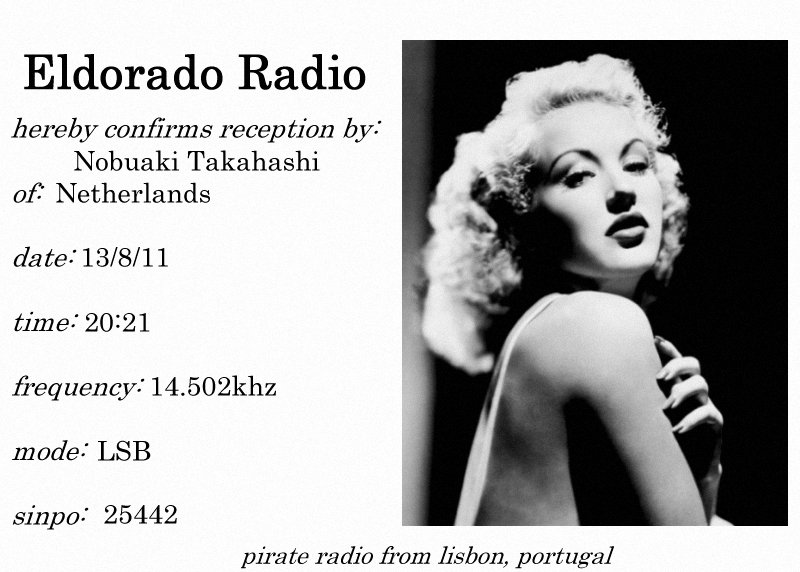The image depicts a black-and-white photo of a young woman on the right side, likely a celebrity from a bygone era, possibly the 1950s. She has curly blonde hair styled in a vintage fashion, and her 1950s-style makeup complements her youthful appearance. She is dressed in a white outfit, and her dark-colored, perhaps red, fingernails grasp her arm as she gazes over her shoulder directly at the camera, with a spotlight illuminating her against a black background. On the left side of the image, there is text in black stating "El Dorado Radio hereby confirms reception by Nobuaki Takahashi of the Netherlands." Below this, details such as date, time, frequency, mode, and SINPO ratings are provided. At the bottom, it reads "Pirate Radio from Lisbon, Portugal."